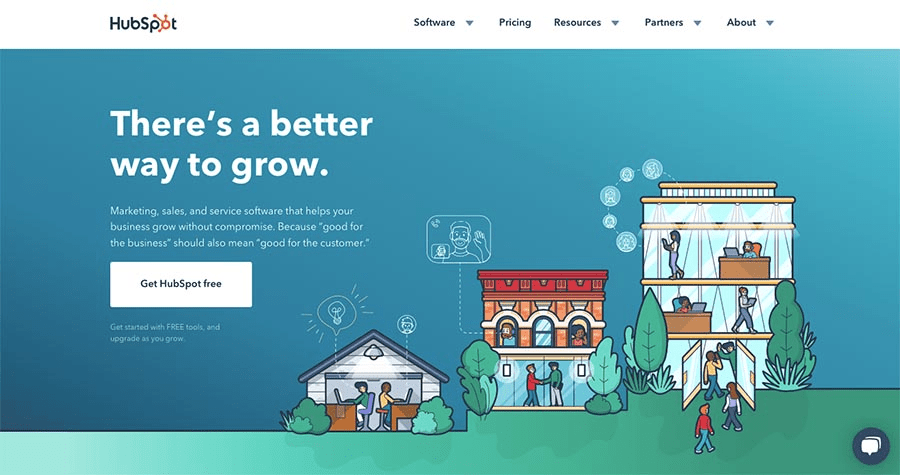At the top left of the image, there is the "HubSpot" logo, while the top right features large dropdown menus labeled "Software," "Pricing," "Resources," "Partners," and "About." Below this, an illustration unfolds against a backdrop of blue sky. 

On the left side of this landscape, a small, garage-like building is depicted, with two individuals inside working on laptops. Adjacent to this, a multi-story building appears, the bottom floor resembling a store while the upper floors look like apartments. In front of this building, two people are seen shaking hands. 

To the right of this scene stands a large, multi-story glass building. The illustration shows people seated at desks inside, as well as others entering and exiting the building. A grassy area extends in front of this modern structure.

In the foreground on the left side of the image, there's a block of text stating, "There's a better way to grow. Marketing, sales, and service software helps your business grow without compromise, because good for the business should also mean good for the customer." Below this text, a white box contains the call-to-action, "Get HubSpot free."